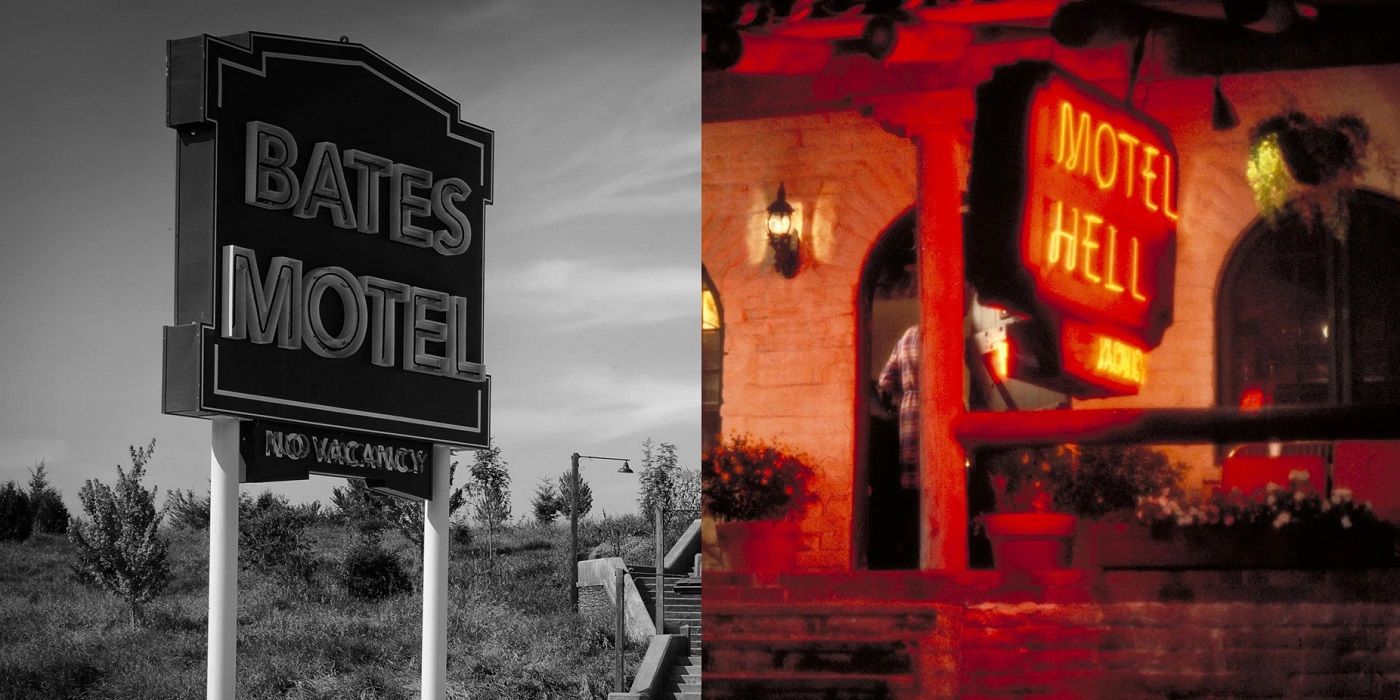This is a collage of two photographs placed side-by-side. The left photograph is a black-and-white daytime image of a Bates Motel sign mounted on two posts, featuring metal lettering with neon tubes spelling out "Bates Motel." Below it, a smaller sign reads "No Vacancy." The scene includes a grassy hill with shrubs, a streetlight, and an outdoor staircase leading up the hill. The background presents a somewhat scrubby landscape. The right photograph, in color and taken at nighttime, shows an old white brick building with an arched doorway and stone steps leading to it. The illuminated neon sign above the entrance reads "Motel Hell" and "Vacancy" in red. The entrance area is adorned with several potted plants on a small porch, bathed in the glow of the neon sign and ambient lighting from the background.